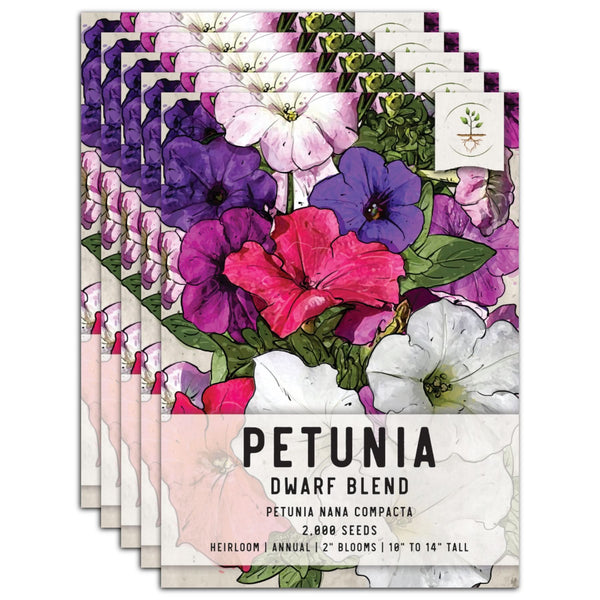The image depicts a stack of five packets of flower seeds, arranged in a staggered, left-to-right pattern against a white background. Each square-shaped packet, made from paper or cardboard, prominently features an illustrated label of different colored Petunia Dwarf Blend flowers, showcasing white, red, blue, pink, purple, and white flowers with a yellow center. The front packet displays detailed information, stating "Petunia nana compacta, 2,000 seeds, heirloom, annual, 2-inch blooms, 10 to 14 inches tall." A logo in the top right corner depicts a plant with visible brown roots and green leaves.